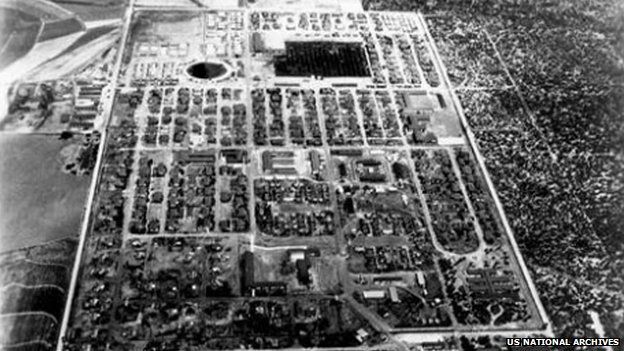This is an aerial black-and-white photograph, likely sourced from the U.S. National Archives, depicting what appears to be a government facility or lab. The image shows a prominent large circular structure on the left side and a large building on the right. The facility is surrounded by a sizable wall, with numerous houses scattered around the area. To the right, there appear to be some trees, and to the left, it looks like open fields. The lack of detail makes it hard to ascertain the exact nature of the site, but its archiving by the U.S. National Archives suggests its significance.